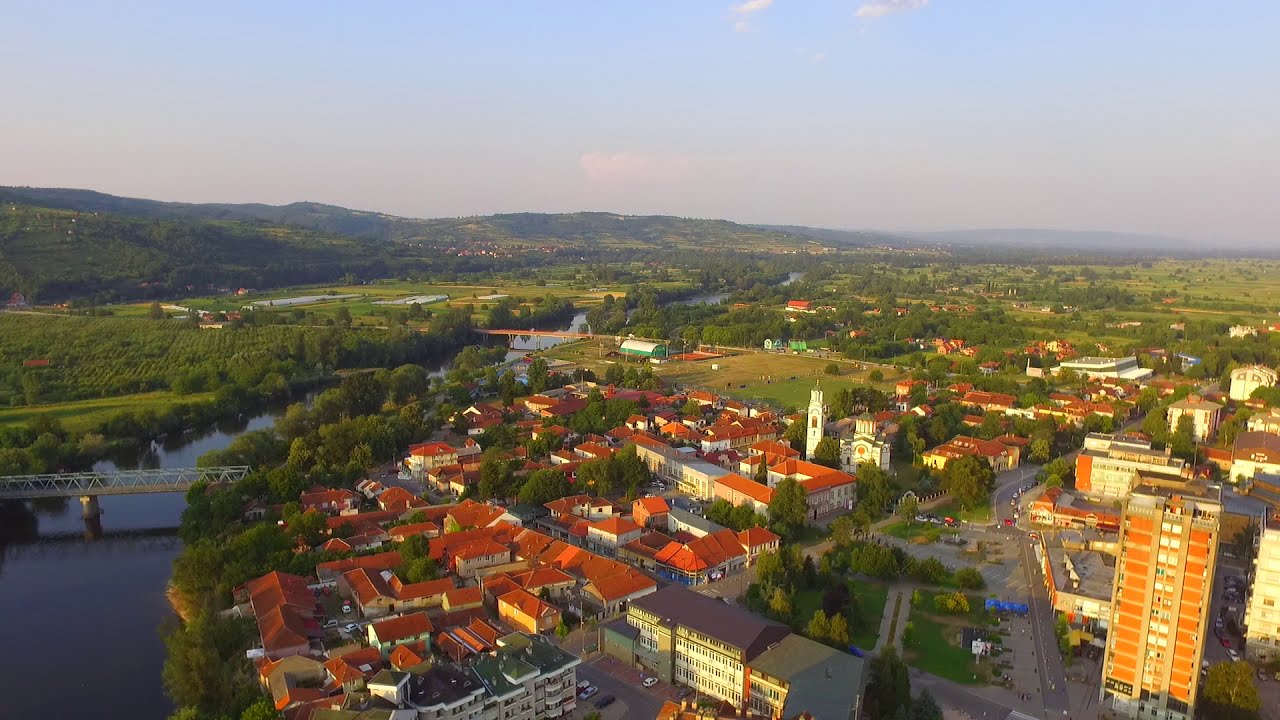An aerial photograph captures a small town with a distinctive mix of natural and urban elements. In the lower right section, a collection of buildings can be seen, featuring a mix of orange and cement structures, as well as homes with reddish clay roofs interspersed with white buildings topped with gray roofs. Dominating the center of the image, a winding river flows from the bottom left corner towards the horizon, crossed by a few bridges. The river divides the scene, with the right bank bustling with roads, buildings, and greenery, while the left bank remains more open, featuring grassy areas and clusters of bushy trees. The backdrop includes rolling green hills and, to the far left, some mountainous terrain. The sky occupies the upper fourth of the image, appearing blue with a slight haze and dotted with clouds, providing a serene canopy over the picturesque landscape below.